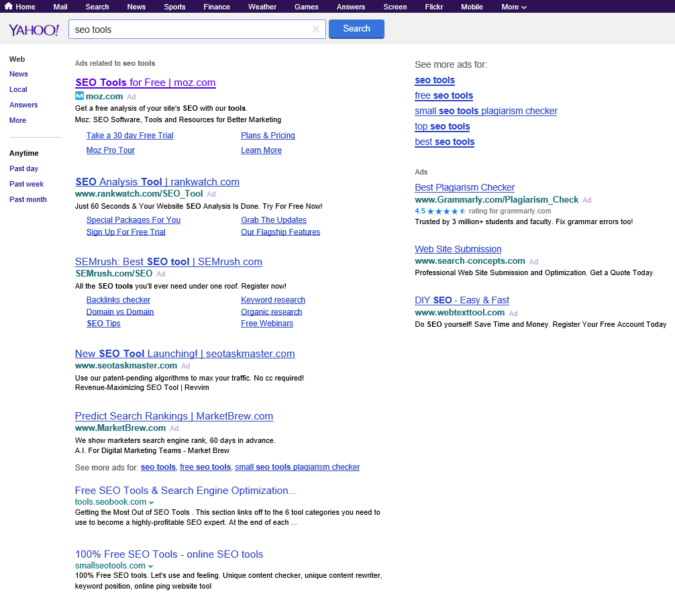In this image, you see Yahoo's search engine interface displaying search results for "SEO tools." The top four results are marked as ads, each offering various SEO-related services. 

1. The first ad is from Moz, promoting "CEO Tools for Free" and promising a complimentary site analysis. Their description mentions access to a suite of SEO software tools and marketing resources (moz.com).
2. The second ad, from RankWatch, offers a "CEO Analysis Tool." It highlights a quick, 60-second website analysis available for free (rankwatch.com).
3. The third ad, from SEMrush, claims to be the "Best SEO Tool." It advertises an all-encompassing SEO toolset under a single platform, inviting users to register (SEMrush.com).
4. The fourth ad, from SEOtaskmaster, introduces a "New SEO Tool Launching." This ad promotes their unique algorithm, designed to boost website traffic with minimal technical knowledge required, and emphasizes its revenue maximizing capabilities (SEOtaskmaster.com).

Each ad includes a mix of URL links and enticing offers to attract users looking for SEO solutions.